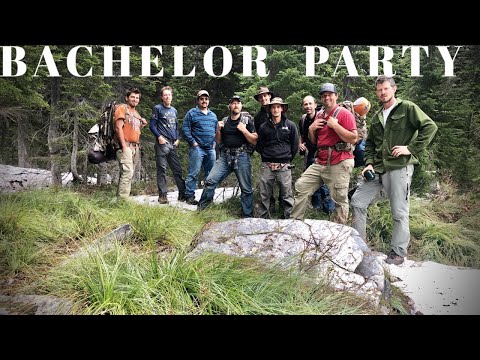A group of nine men stand together on a white sandy trail, dressed in casual hiking attire consisting of either jeans or beige cargo pants. Some of the men carry camping packs, while others are just posing for the photo. They are surrounded by tall, dry green grass, with a prominent white boulder in the foreground and dense pine trees in the background. The men are all looking directly at the camera. The image is framed with large black borders at the top and bottom, giving it a theatrical feel. Above their heads, in bold white letters, the words "Bachelor Party" are displayed.